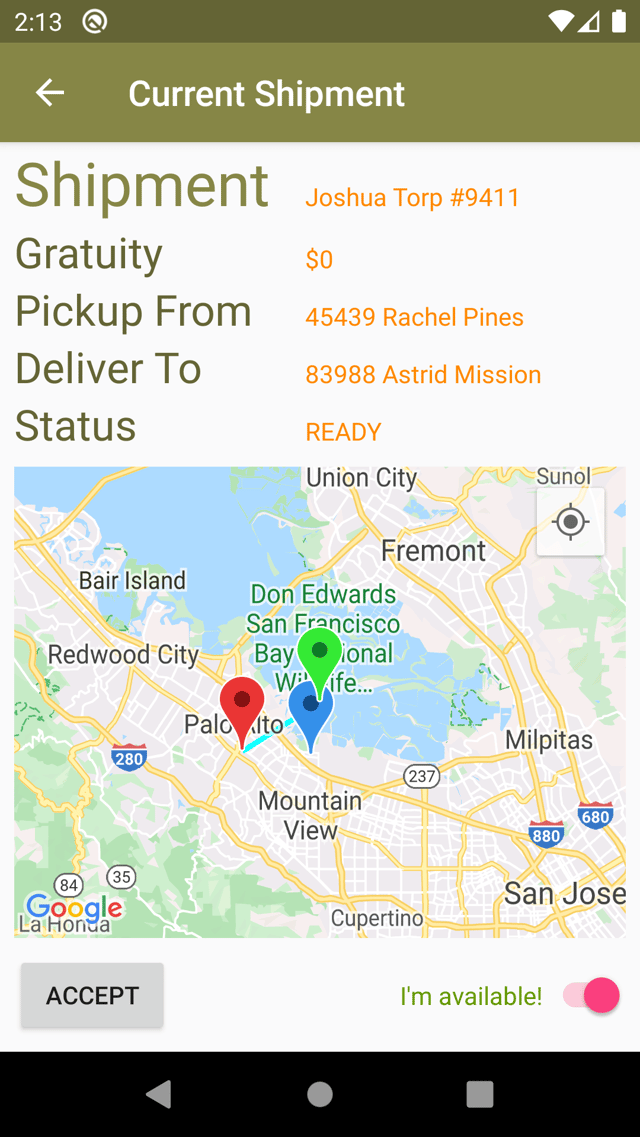This mobile screenshot captures a web page titled "Current Shipment," displayed in a dark olive green header with a medium olive green subheader. The top left features the time, while the top right showcases Wi-Fi and battery icons. Below the header lies essential shipment details in a large green font, organized under five categories: 

- **Shipment**: Destined for Joshua Torp, shipment number 9411.
- **Gratuity**: 0
- **Pickup From**: 45439 Rachel Pines
- **Deliver To**: 83988 Astrid Mission
- **Status**: Ready

Directly below this information, a Google map is displayed, marked with three location indicators in red, green, and blue, along with visible interstates. A gray "Accept" button is positioned beneath the map, alongside an "I'm Available" slider, which is currently turned on. The footer blends seamlessly with a black background featuring three gray icons. The overall image provides a comprehensive view of the current shipment status, including the complete addresses for pickup and delivery, map coordinates, and readiness status, all within a user-friendly interface.